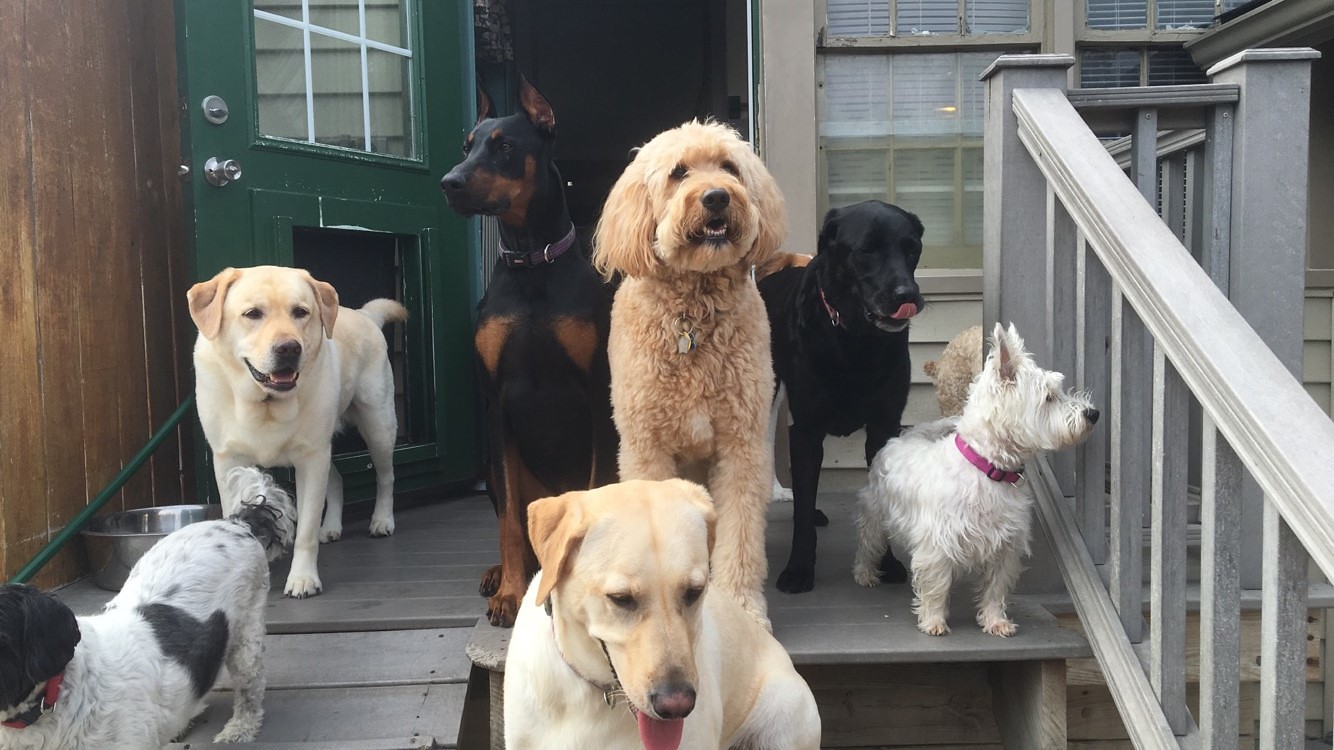In this photograph, we see a back porch scene bustling with canine activity. The gray steps of the porch are accompanied by a gray ramp to the left. On the porch, there are seven dogs of varying breeds, all either sitting or standing, and facing outward toward the camera as if they are eagerly observing their surroundings. The group includes two yellow Labradors, a Doberman, a small white Scotty, a black Poodle mix, a likely black Labrador, and a black and white spotted dog, which might be a shaved-down Lhasa Apso.

The porch floor is made of wooden boards, and a large silver bowl is placed on it. The background features a dark green door, distinguished by its window with white molding, that opens inward toward the house. A hint of indoor blinds can be seen through the doorway. To the left of this green door, there appears to be a wooden fence, and possibly a doggy door at the bottom. On the right side of the porch, there is a banister painted white which lines the steps. The scene overall encapsulates a serene yet vibrant gathering of diverse dogs on a typical suburban porch.